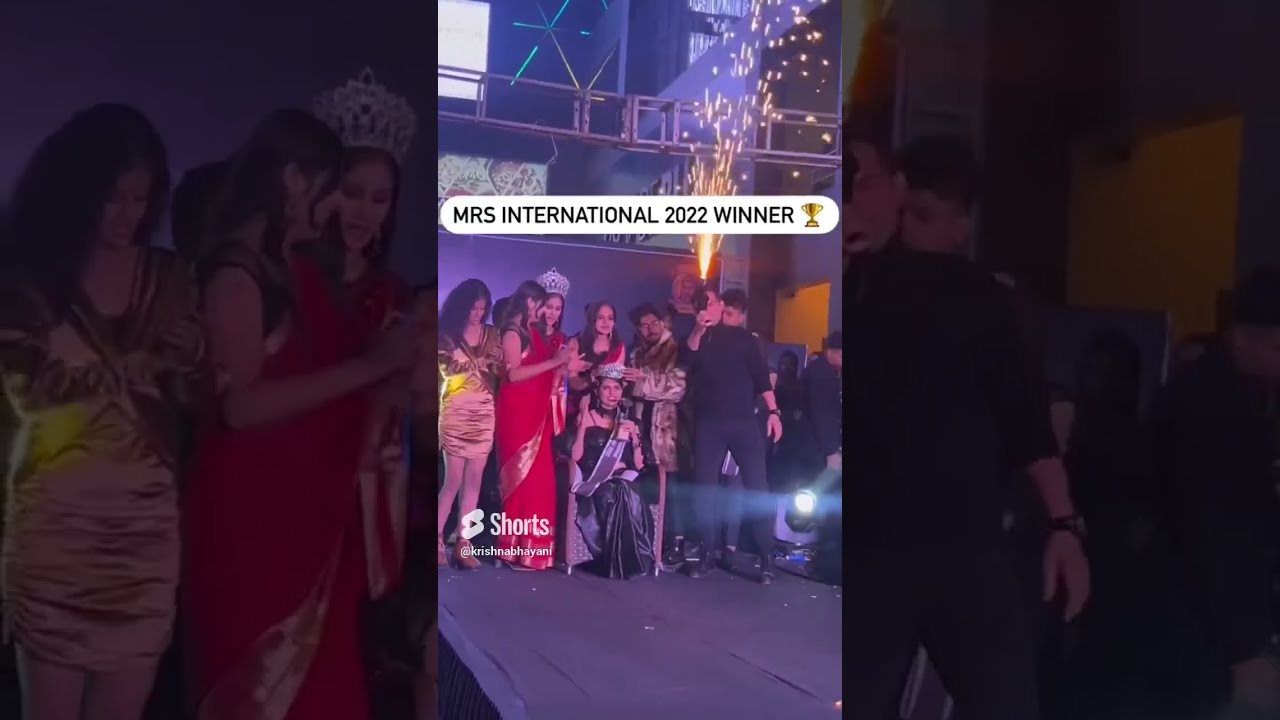The image is a screen capture of a YouTube short or social media reel, showcasing a moment from the Mrs. International 2022 awards ceremony. The center panel, brighter than the darkened left and right panels, features a group of around ten people on stage. The focal point is a woman in a black dress and sash sitting at the front while another person places a crown on her head, indicating her as the winner. Around her, several other women in dresses applaud. A man dressed in an all-black outfit is seen holding a sparkler or firework, adding to the celebratory atmosphere. The background includes scaffolding and a screen, with someone holding a spotlight to illuminate the scene. Dominant colors in the image are red, gold, and black, with some gray, blue, and green tones. The top part of the image has a banner stating "Mrs. International 2022 winner," accompanied by a trophy emoji. A watermark in the bottom left corner identifies the content creator as Krishna Bhayani (K-R-I-S-H-N-A B-H-A-Y-A-N-I), along with a play button icon indicating its origination from a YouTube short.